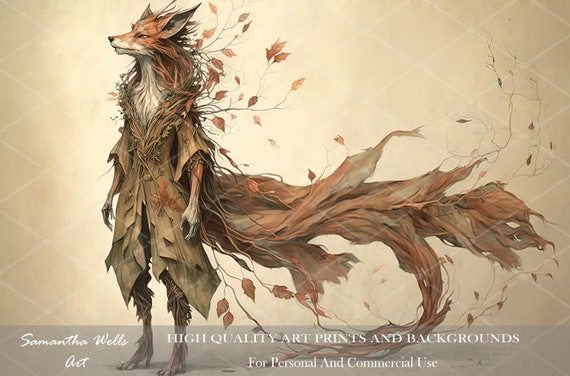In this rectangular, full-color illustration set against a golden beige background, a human-animal hybrid figure stands upright, merging both fox-like and human characteristics. The creature features a fox's head turned westward, adorned with scraggly brown fur. Its emaciated arms and legs terminate in hoof-like feet, contributing to its surreal appearance. Draped over its form is a cloak that resembles a large leaf, rendered in rich brown hues and seemingly caught in a gust of wind, sweeping dramatically from the creature’s back. Below the image, in crisp white print, the text reads, "Samantha Wells Art," followed by, "high-quality art prints and backgrounds for personal and commercial use."